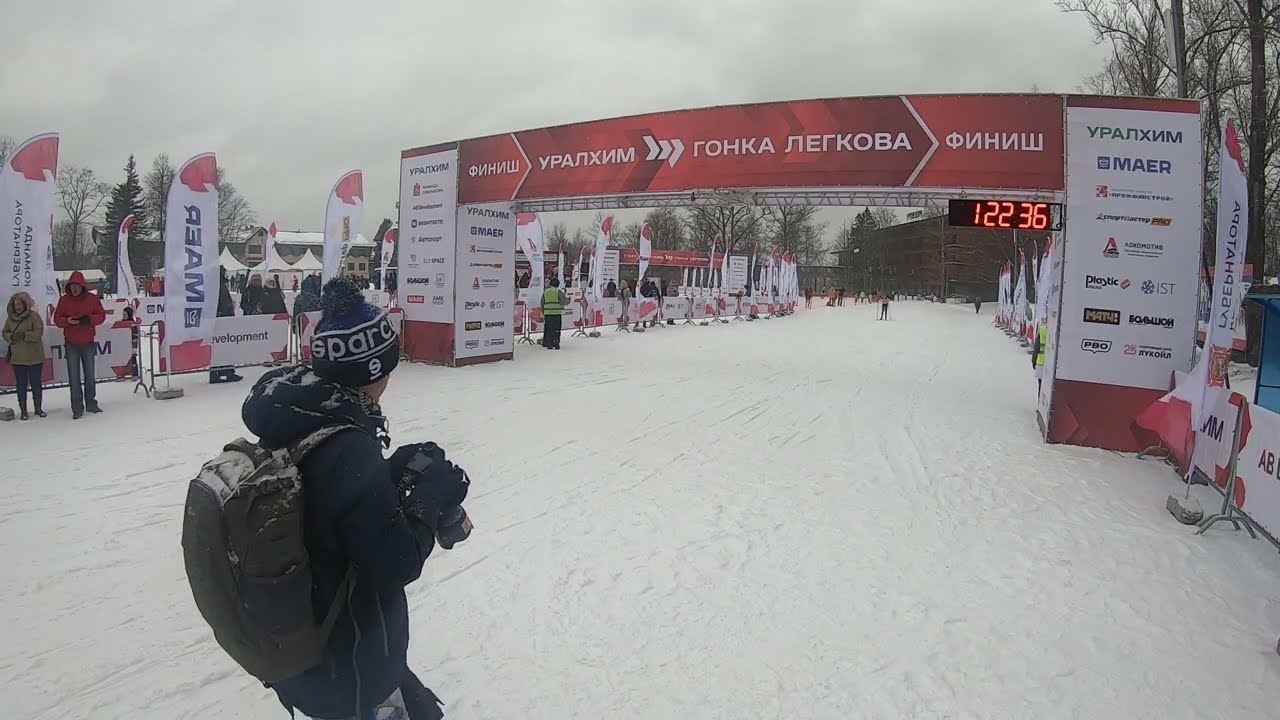The image captures a vibrant scene at a ski race finish line on a snowy, overcast day. In the foreground, a young photographer wearing a navy blue beanie with "SPARC" written on it, a matching blue jacket, and a grayish-brown backpack stands with a camera poised, ready to capture the imminent arrival of skiers. The figure is slightly turned to the side, providing an almost profile view as they focus on the action ahead. The snowy ground is interspersed with colorful fencing and banners in a foreign European language, indicating numerous sponsors and adding to the international atmosphere of the event. Dominating the center of the image is a red and white archway finish line supported by scaffolding, featuring a visible digital timer displaying "1:22:36." Spectators and officials line the sides of the course, creating a bustling backdrop as they await the racers. In the distance, a skier can be seen rapidly approaching the finish line, framed by the stark, leafless trees under a cloudy winter sky, completing this dynamic and detailed scene.